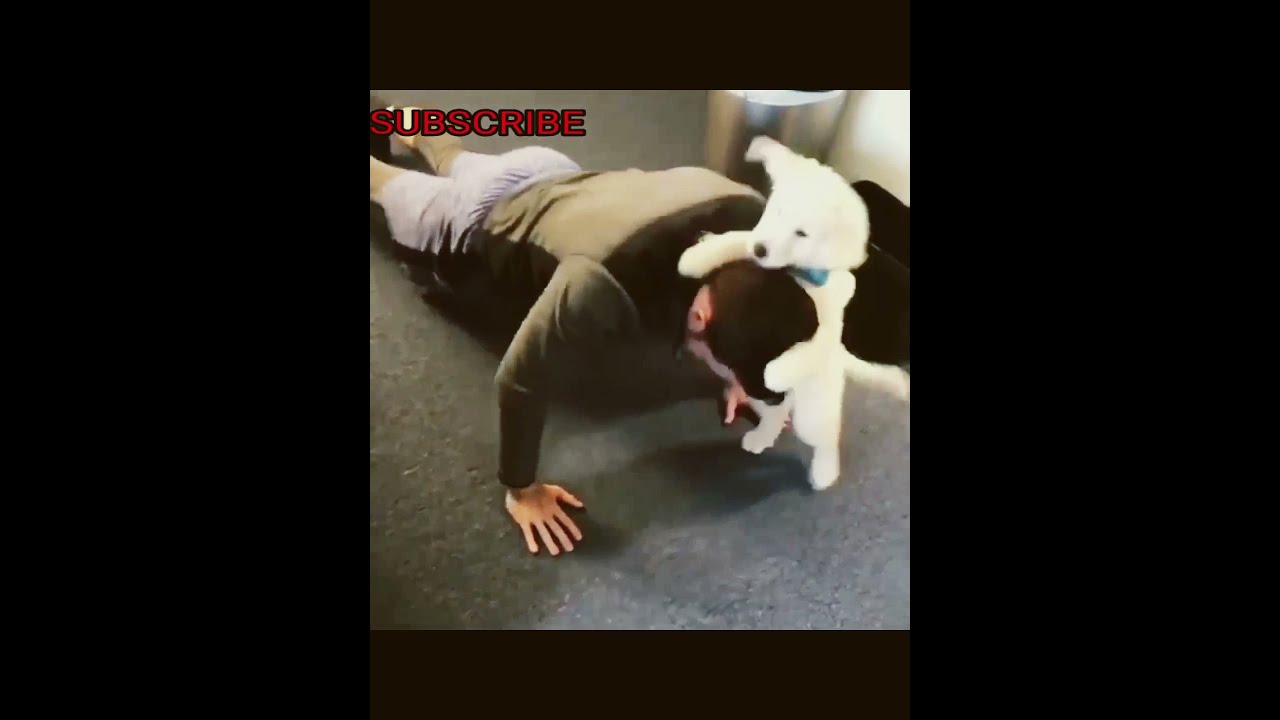In this screenshot from a YouTube video, a man with dark hair and possibly a beard is seen performing a plank exercise. He is dressed in gray track pants and an olive green long-sleeve shirt with black trim around the neck. The setting appears to have a gray carpet or gym mat floor, with a blurry silver trash can and a tan wall in the background, suggesting an indoor environment. Dominantly, a white puppy with a blue bow perched atop its head has leaped up and placed its front paws on the man’s head and neck, as if trying to hold on. The puppy’s playful eyes and nose contrast with the man’s focused posture. The entire scene is bordered by black vertical bars on the sides and dark brown horizontal bars at the top and bottom. In the top left corner of the image, the word “SUBSCRIBE” is prominently displayed in red letters with a black outline.